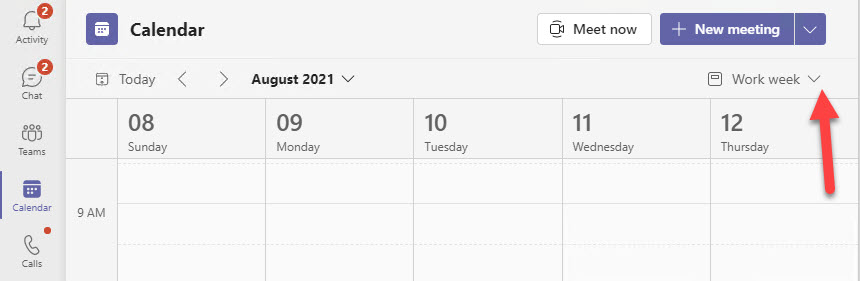A detailed screenshot of a Calendar app interface is displayed. On the right-hand side of the screen, there's a vertical sidebar featuring various icons: a bell for activity notifications, a word bubble for chat, stylized people representing Teams, a calendar icon for the Calendar view, and a phone icon for calls. The Calendar page is currently selected. At the top of the interface, a header in black text against a gray background reads "Calendar." Next to this, there are options to "Meet now" or "Add a new meeting." Just below the header, the month "August 2021" is displayed, indicating that the current view is for the week of Sunday the 8th to Thursday the 12th. The app appears to be designed for team management, enabling coordination and scheduling within a team environment.